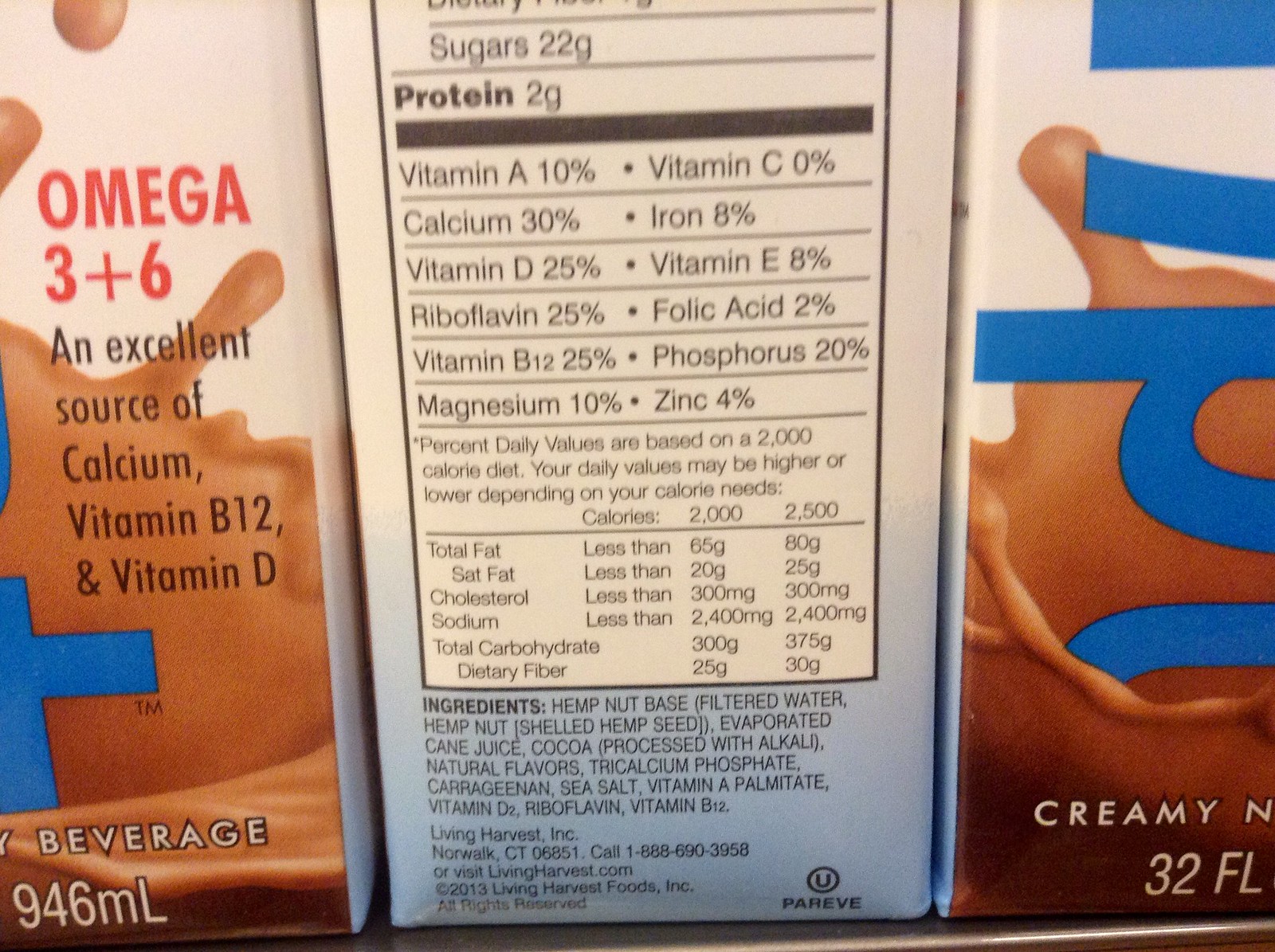This image showcases the backside of a milk beverage container, highlighting its nutritional information. To both the left and right of the label, the design elements of the product's front side are visible. On the left side, the container features the words "Omega 3 & 6," "An excellent source of calcium, vitamin B12, and vitamin D," and "946 milliliters." The beverage appears to be chocolate milk, evidenced by the depiction of a rich brown liquid on the container's artwork. The center of the image focuses on the vitamin label, detailing various percentages of essential vitamins and listing the ingredients below. On the right side, the container reads "creamy" at the bottom, along with "32 FL," indicating fluid ounces.